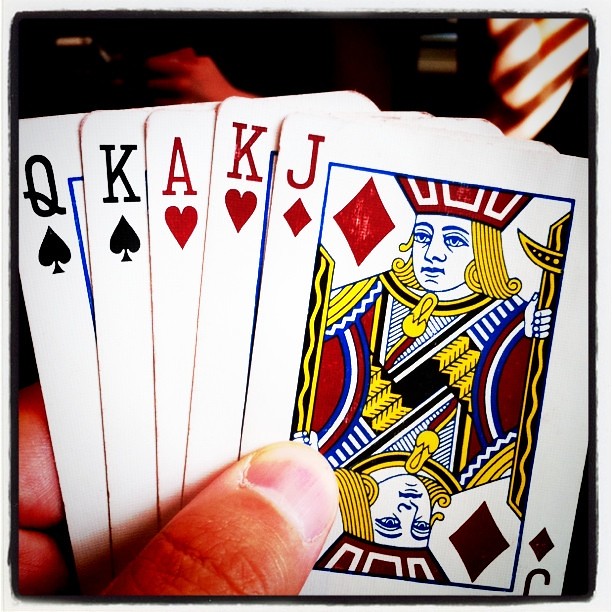In this image, the background features a blend of black and reddish hues. In the upper right corner, a window blind is visible with light filtering through its slats, casting a reddish-yellow glow intersected by black lines. In the lower left-hand corner, a person with a medium complexion is holding five playing cards. Their thumb and four fingers are clearly seen grasping the cards. From left to right, the cards are as follows:
1. The Queen of Spades, with the black "Q" and spade symbol.
2. Part of a blue box is visible next to the Queen of Spades.
3. The King of Spades, featuring the black "K" and spade symbol.
4. The Ace of Hearts, marked with a red "A" and heart symbol.
5. The King of Hearts, displaying the red "K" and heart symbol.
6. The Jack of Diamonds, depicted with the red "J" and diamond symbol, and an image of the Jack with his head oriented both at the top and bottom alongside the diamond symbol.